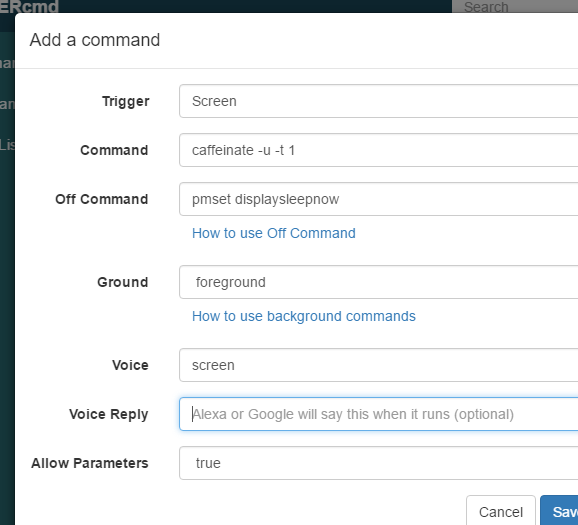A detailed caption for the described image could be:

"This image is a partial screenshot of a web interface designed for setting up voice commands. The interface is predominantly white with a black bar along the top and left edges, seamlessly blending into the background on the right and bottom sides. At the very top of the interface, there is a header that reads 'Add a Command'. Below this header, a series of configurational options are displayed in an organized list. 

The first option is labeled 'Trigger' with an adjacent rectangular input box that currently reads 'Screen'. The second option is 'Command,' with the input box showing 'caffeinate-u-t1'. Moving down, the 'Off Command' field has 'pm set, display sleep now' written inside its corresponding box. 

Following these options, there is a blue hyperlink reading 'How to use off command,' indicating a clickable instructional link. Below this link, the 'Ground' option is set to 'Foreground'. Another blue hyperlink beneath this reads 'How to use background commands,' providing additional clickable guidance.

The 'Voice' field is also set to 'Screen', and the 'Voice Reply' field contains a placeholder text: 'Alexa or Google will say this when it runs, optional'. Lastly, there is a 'Allow Parameters' field set to 'True'. 

At the bottom of the interface, side-by-side buttons labeled 'Cancel' and 'Save' are available for managing the configuration."